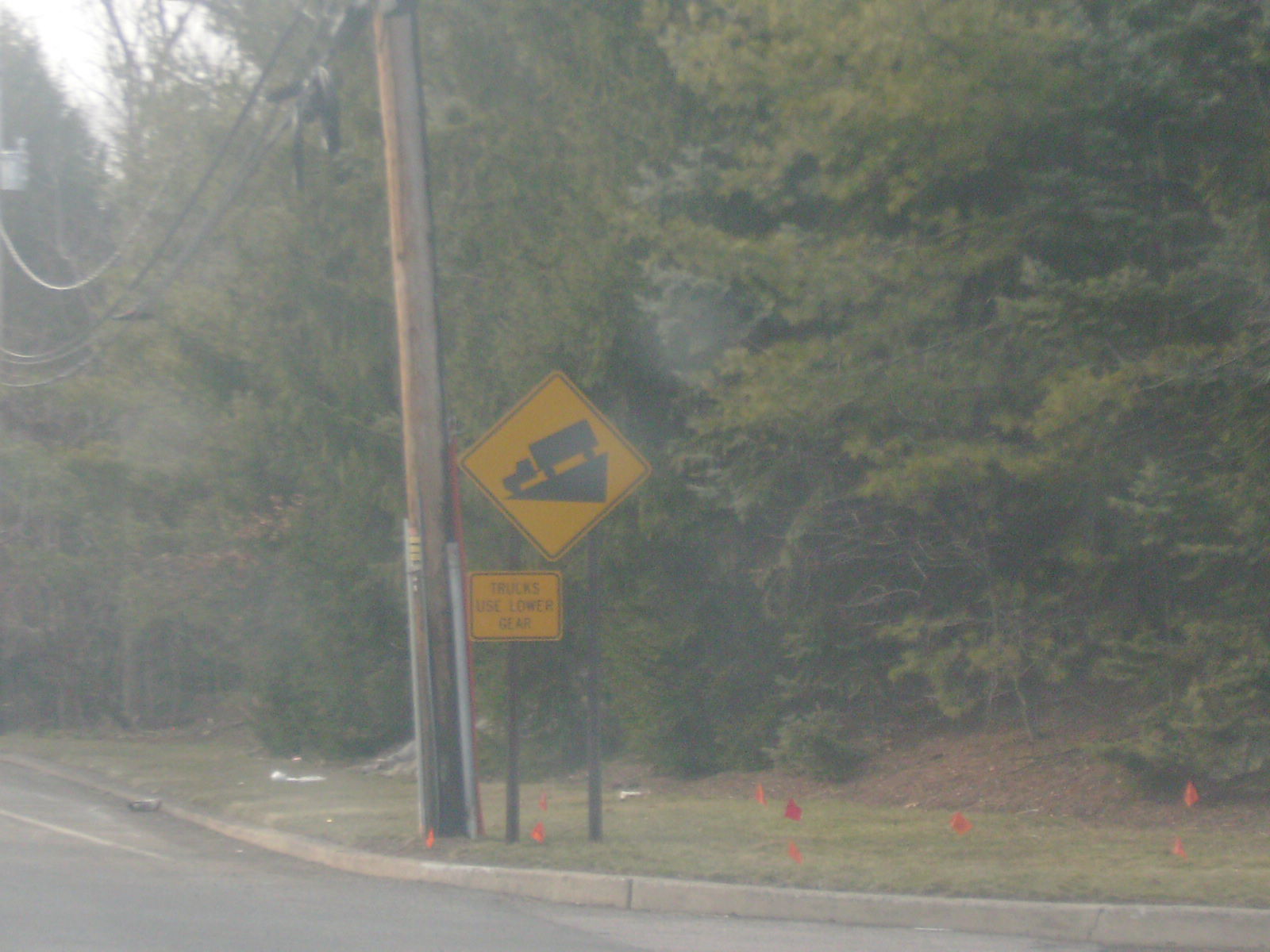This photograph, seemingly taken through a pane of glass or enveloped in a subtle white haziness, depicts a charming corner of a street. At the bottom, a grey paved road curves gently to the left, bordered by a neat curb. On the left side of the image, a tall brown telephone pole stands, with electric wires stretching outward and disappearing off the frame. The background is dominated by a thick grove of towering pine trees, providing a natural backdrop. Scattered around the grassy area near the curb are small red or orange flags, adding a splash of color. Prominently positioned are two yellow road signs: one displaying the image of a truck descending a slope, and the other instructing, "Trucks Use Lower Gear."